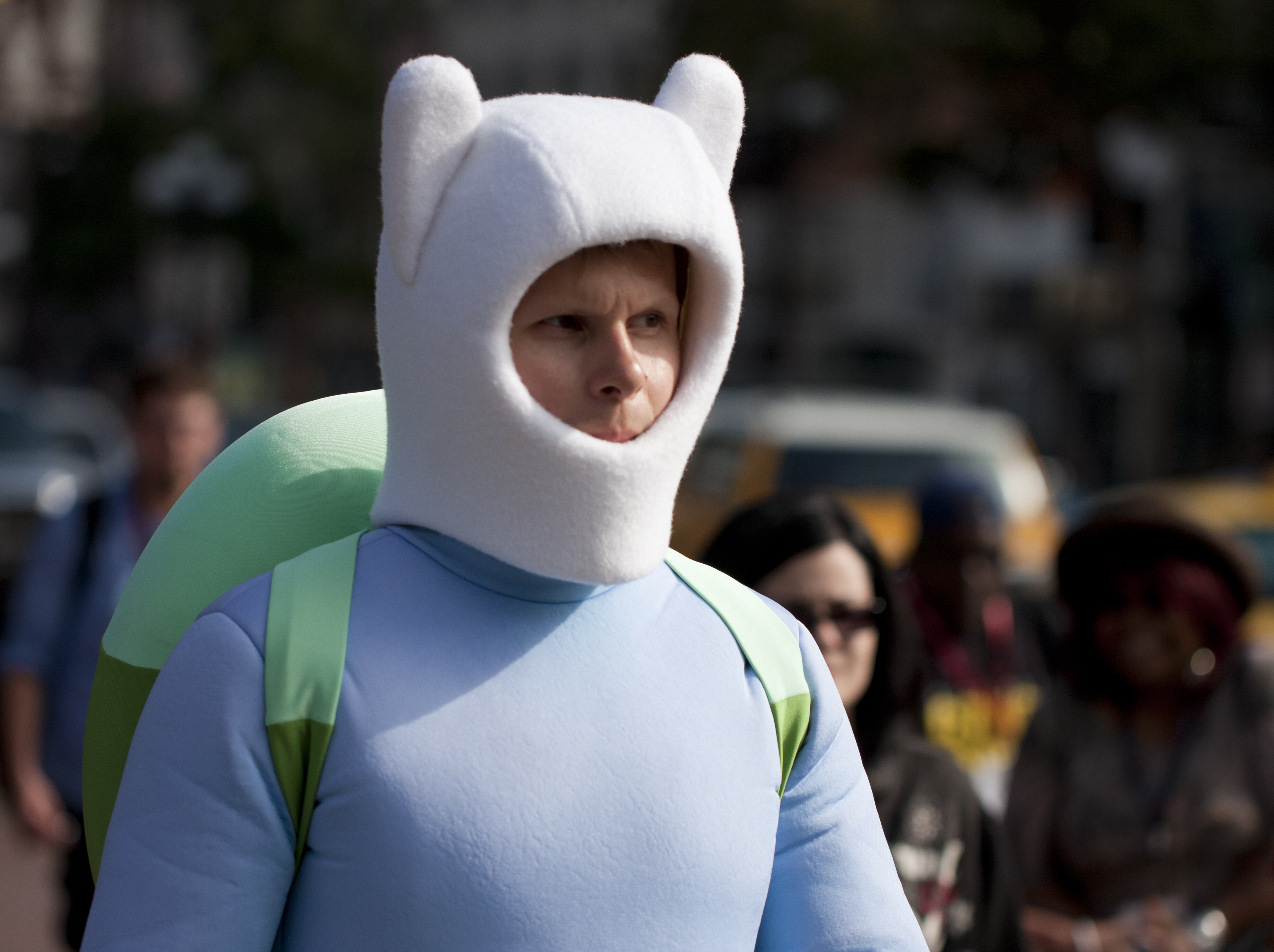The photograph captures a candid moment of a Caucasian man at what appears to be a convention, possibly dressed in cosplay inspired by the cartoon show Adventure Time. The man is wearing a distinctive outfit that includes a puffy, white, full-coverage hat with prominent ears, giving him a playful, almost childlike appearance. His attire features a light blue padded shirt with long sleeves, hinting at some kind of costume. On his back, he carries a two-toned green backpack, with a light green top and a darker green bottom. The background is blurred but reveals other people, some wearing lanyards and others smiling, adding to the lively atmosphere of the event. The man looks off to the right, not directly engaging with the camera, enhancing the candid nature of the shot.